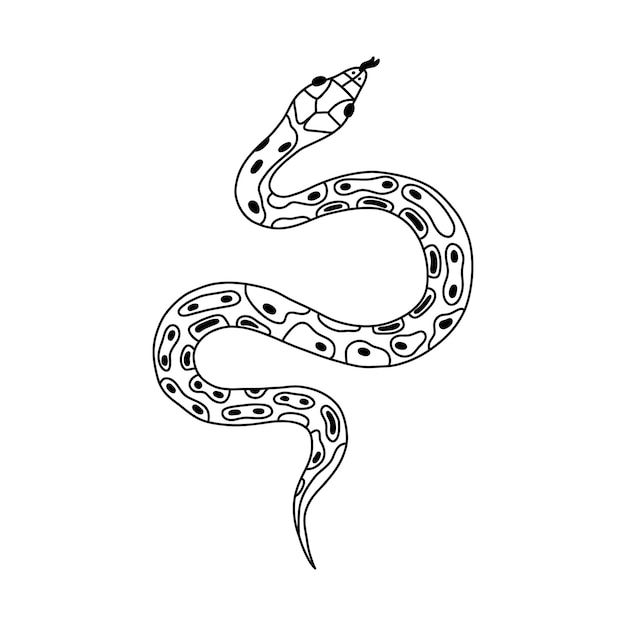This image depicts a detailed, line-drawn snake set against a white background, giving it the appearance of a coloring book illustration. The snake begins with its head positioned at the top right and continues to coil down into its tail at the center bottom. The head of the snake features two black eyes and a forked black tongue protruding from a mouth flanked by two small nostrils. Distinct markings cover the snake's entire body, starting with five segmented sections on its head. These irregular, peanut-shaped patterns are distributed along the length of the snake, enclosing varying numbers of black dots—ranging from none, two, usually one or two, and occasionally several in each pattern. Prominently near the neck, one larger segment contains four distinct black dots. The snake's body curves twice in a traditional serpentine S-shape before tapering off into its tail, which has a distinct marking near the tip that is just outlined without any black dots inside. This juxtaposition of outlined forms and dotted patterns gives the snake a richly detailed and visually intriguing appearance.